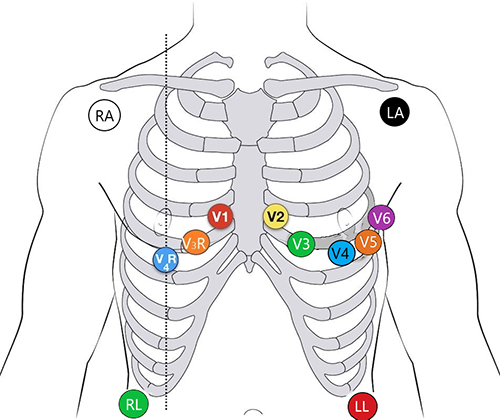The illustration is a detailed, computer-aided anatomical animation of a male torso, focusing particularly on the skeletal structure of the chest. The torso is depicted from the midsection of the neck down to the belly button, and includes outlines of the upper arms and shoulders. The central feature is a transparent view of the ribcage, meticulously labeled with various colored circles that serve as keys for identifying different ribs and other parts of the ribcage. 

Each section of bone in the ribcage is marked with distinct labels ranging from V1 to V6, each represented by a different color: V1 (red), V2 (yellow), V3 (green), V4 (blue), V5 (orange), and V6 (purple). Additional labels include RA (white) and LA (black) at the top, as well as RL (green) and LL (red) at the bottom. This labeling system appears to categorize and identify specific bones and sections within the ribcage, contributing to the comprehensive educational value of the diagram.